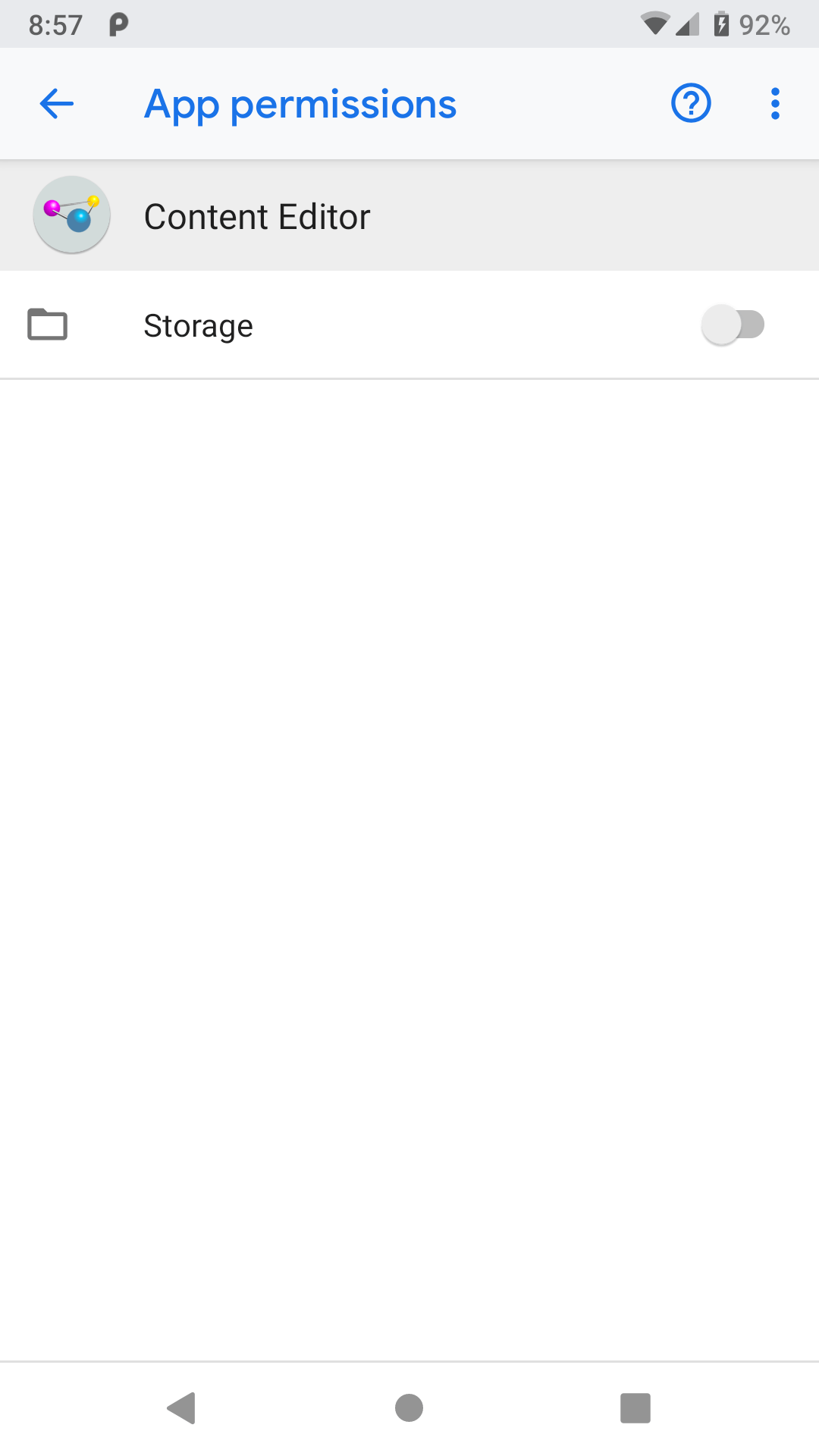This is a detailed screenshot displaying app permissions on a cell phone with a primarily white background. 

At the top of the screen, a faint light gray rectangle spans the full width from left to right. In the top left corner of this rectangle is the current time, "8:57 PM," displayed in black text. Moving toward the right end of this rectangle, icons appear sequentially: a Wi-Fi indicator, connectivity bars, and a battery symbol displaying "92%".

Below this, a larger light blue-gray rectangle, also stretching from left to right, features blue text. On the left side of this rectangle is a back arrow icon pointing to the left, followed by the label "App permissions." At the right side are an outlined blue circle with a blue question mark inside and three vertical blue dots.

Further down, there is another light gray rectangle, slightly darker than the previous one, extending from left to right. On its left side sits a darker gray circle containing three small, colored circles: pink, blue, and yellow. To the right of this circle, black text reads "Content Editor."

Below this area, the background returns to white, displaying a small file icon on the left, followed by the text "Storage." To the far right within this section is an on-off toggle switch, which is currently toggled off.